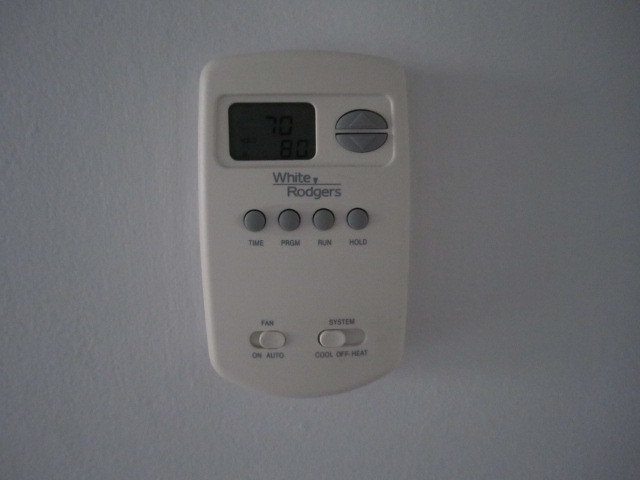A close-up image showcases a White-Rodgers thermostat mounted on a white wall. The thermostat itself is white with a rectangular shape, featuring rounded edges at the bottom and squared edges at the top. At the bottom of the thermostat are two switches: a 'Fan' switch with 'On' and 'Off' options, and another switch with similar 'On' and 'Off' options to its right. Moving upward, four small gray buttons are visible, though the text labeling them is difficult to read due to its small size. Above these buttons, the White-Rodgers logo is prominently displayed, followed by a small screen that indicates the thermostat's settings. To the right of the screen, two gray buttons with up and down arrows allow for temperature adjustments. The overall design of the thermostat is sleek and functional, blending seamlessly with its surroundings.